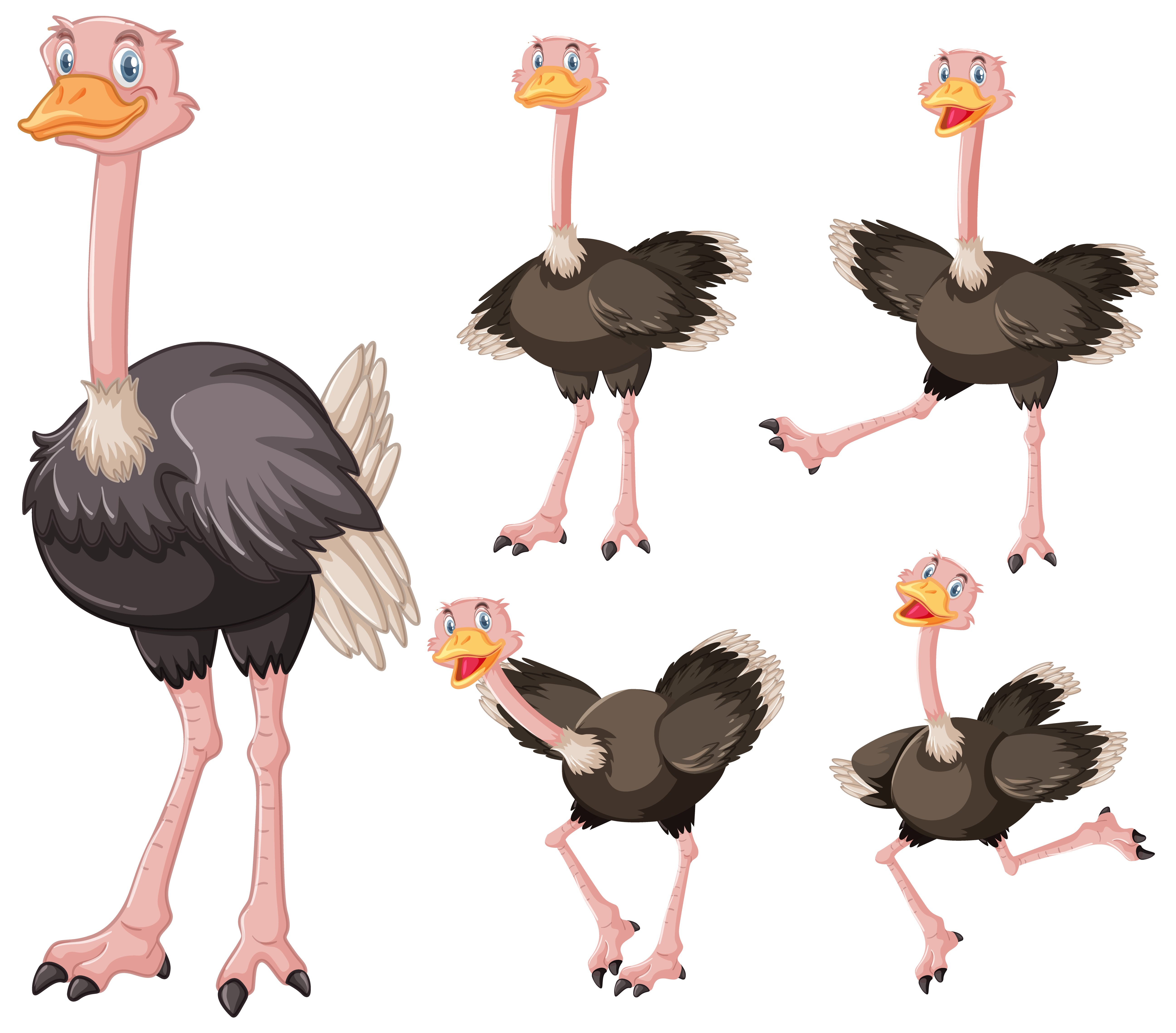This cartoon image features five playful and odd-looking ostriches set against a white background, rendered in a professionally made, comic book style suitable for a kid's show or book. All of the ostriches sport pink heads, necks, and legs, with vivid orange bills and expressive blue eyes. Their bodies are predominantly grey and black with white tips accentuating their feathers. The ostriches are all smiling, exuding a happy demeanor as they seem to be interacting with the viewer.

On the left side of the image, there is a large depiction of an ostrich standing upright with its neck extended. To the right, the remaining four ostriches are grouped together in a dynamic arrangement, forming a two-by-two grid. These ostriches are in various poses that suggest movement and interaction: one is standing, another is kicking its leg to the side, a third is bending forward with its neck outstretched, and the last one is energetically kicking up its leg while flapping its wings. This setup gives the impression that two of the ostriches might be dancing, adding an animated and lively touch to the overall composition.